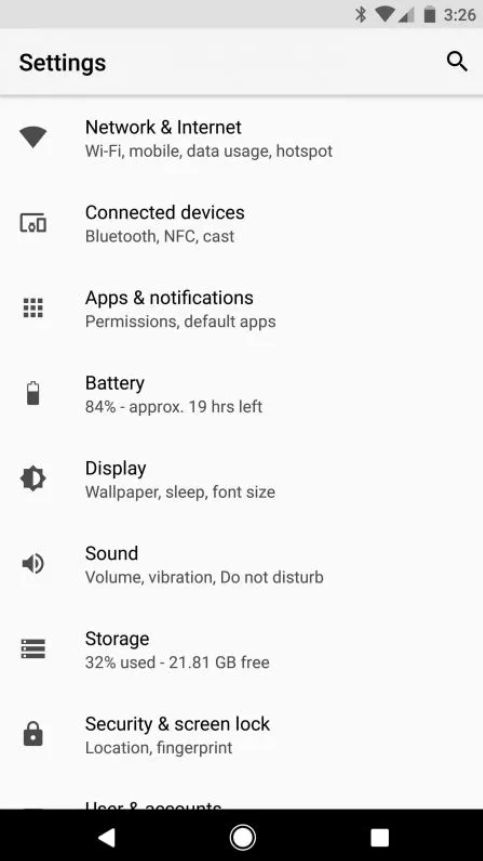A detailed description of the iPhone settings menu screenshot:

The screenshot showcases the settings menu of an iPhone mobile device. The interface is organized into a comprehensive list of options for customizing and managing various aspects of the device. The top of the settings menu features the following categories:

1. **Network & Internet**: This section likely includes options for managing Wi-Fi, cellular data, and other network-related settings.
2. **Connected Devices**: Options under this menu are for pairing and managing Bluetooth devices, as well as other connected peripherals.
3. **Apps & Notifications**: This category would typically encompass options for managing app permissions, notification settings, and recent app activity.
4. **Battery**: The current battery information is prominently displayed here, indicating the battery percentage at **84%** with an estimated **19 hours** of usage remaining. This section also likely includes battery health and usage statistics.
5. **Display**: Adjustments for screen brightness, wallpaper, and other display settings can be found here.
6. **Sound**: This menu allows for the customization of volume levels, ringtone selections, and other audio settings.
7. **Storage**: Provides insights into the storage capacity of the device, detailing how much space is used and what types of files are occupying it.
8. **Security & Screen Lock**: Includes settings for securing the device, such as configuring screen locks, setting up biometric authentication, and managing security protocols.

Each option within the main settings menu allows users to fine-tune the functionality and performance of the iPhone, offering a tailored and optimized user experience.